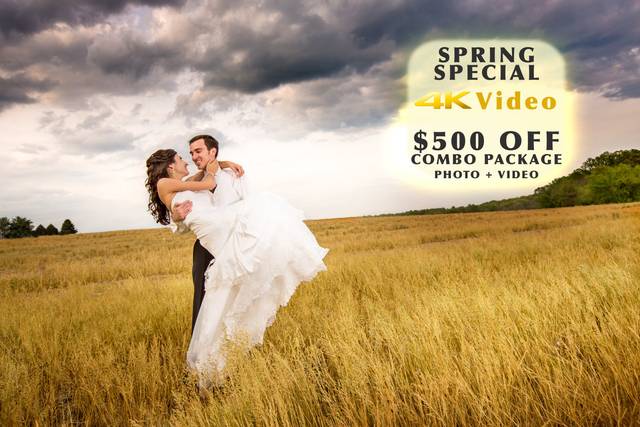The image, an advertisement for a wedding photographer, features a bride and groom in a picturesque field, promoting a "Spring Special 4K Video, $500 Off Combo Package: Photo and Video." The couple, a white pair with brown hair, is captured in a tender moment where the groom, dressed in a suit, carries the bride, who is wearing a strapless wedding gown with her long hair styled half up, half down, in a honeymoon-style embrace. The bride's arms lovingly encircle the groom's neck, and one hand gently touches his face as they smile deeply into each other's eyes. They stand in a knee-high grassy or hay field with trees bordering the scene and an overcast sky that hints at an impending storm, casting a moody yet romantic backdrop. A gold box in the upper-right corner showcases the promotional text, enhancing the special offer's appeal.